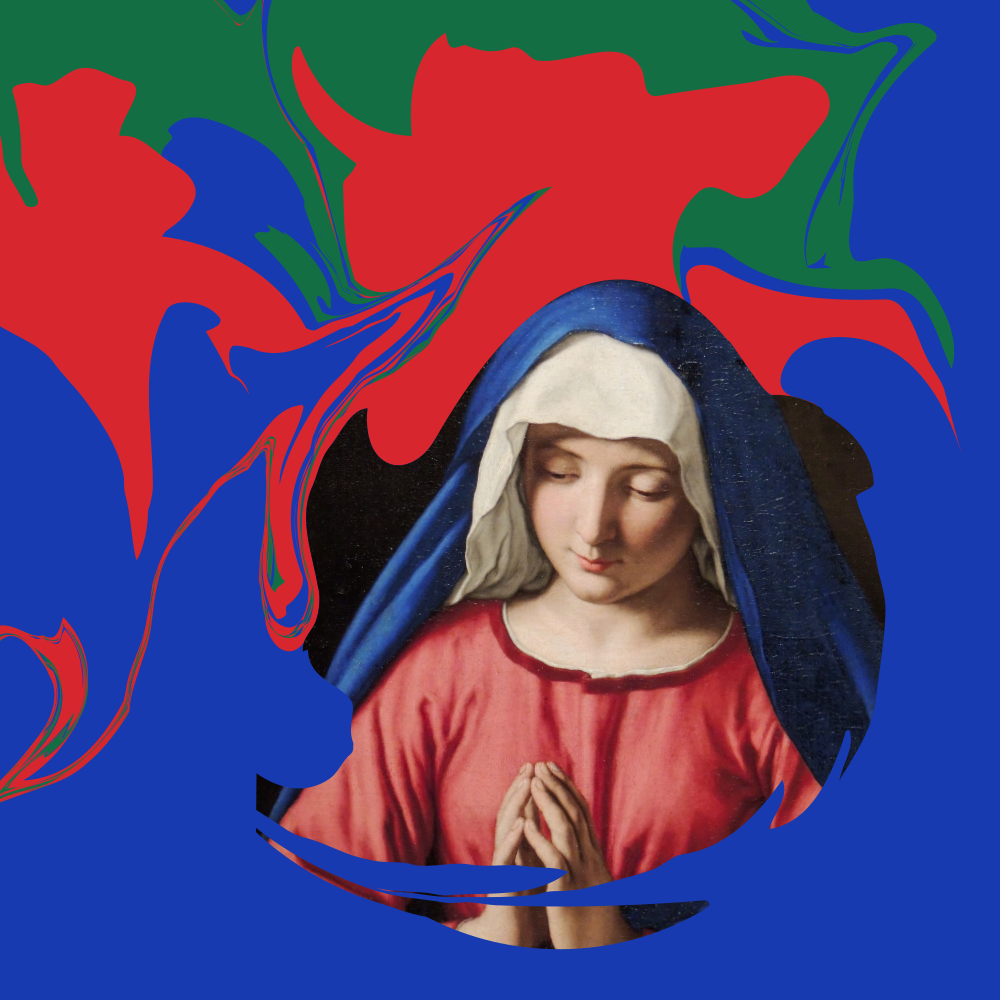The image features a striking juxtaposition of two artistic styles: a central realistic portrayal of the Virgin Mary set against a vibrant, abstract background. The Virgin Mary, depicted in a Renaissance-like style, is clothed in a red tunic and adorned with a white headcloth draped with a blue robe. Her hands are clasped together in a prayerful gesture, and her serene gaze is directed downward. This detailed, grainy depiction of Mary contrasts sharply with the surrounding abstract artwork—a dynamic swirl of matte paint in blue, red, and green. The swirling colors create an almost frame-like effect around her, with the paint predominantly blue on the bottom left and right, and combinations of blue, red, and green swirling around the rest of the image. The background behind Mary is black, adding a stark contrast that heightens the distinct blend of the two artistic styles.